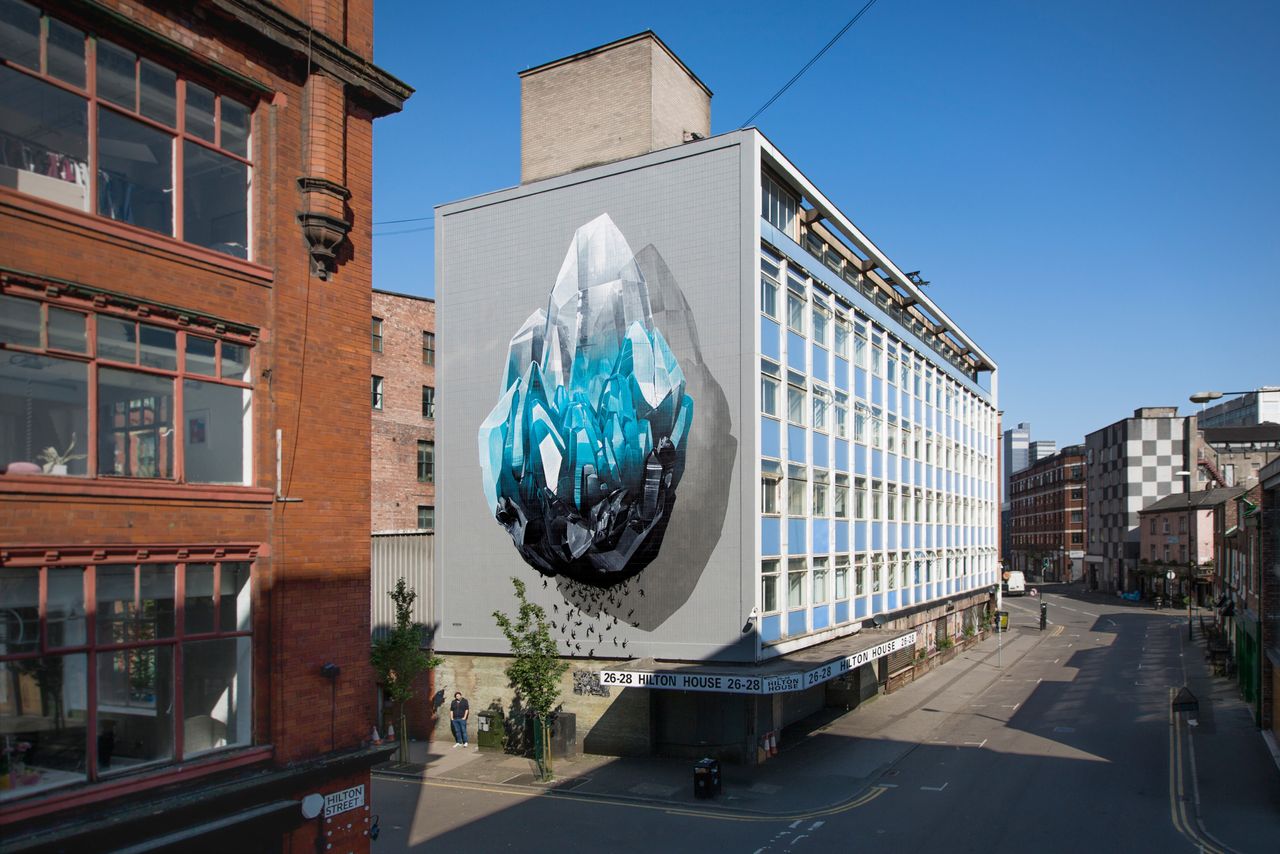The image depicts a bustling city street lined with buildings. On the left, there is a prominent red brick building, featuring four levels including the street level, which has a sign that reads "Hilton Street." The building next to it, central to the image, is a gray structure with five stories above the ground level. This building is notable for the repeated text "26 to 28 Hilton House" along its front.

A striking feature of this gray building is a large mural on its side, depicting a crystal. The crystal artwork displays a gradient from white at the top, transitioning through blue, and finally to black at the bottom. Small black objects or creatures appear to be falling from the crystal, adding a dynamic element to the scene. The sky above is clear blue, casting distinct shadows of the buildings onto the road below.

In the background, various buildings of differing colors and architectural styles can be seen, including more red brick structures and a distinctive checkered-patterned building. The street itself appears mostly deserted, with just a few people on the sidewalk and a single van driving in the distance. The detailed portrayal of the buildings, shadows, and clear sky contribute to the vibrant depiction of this urban setting.